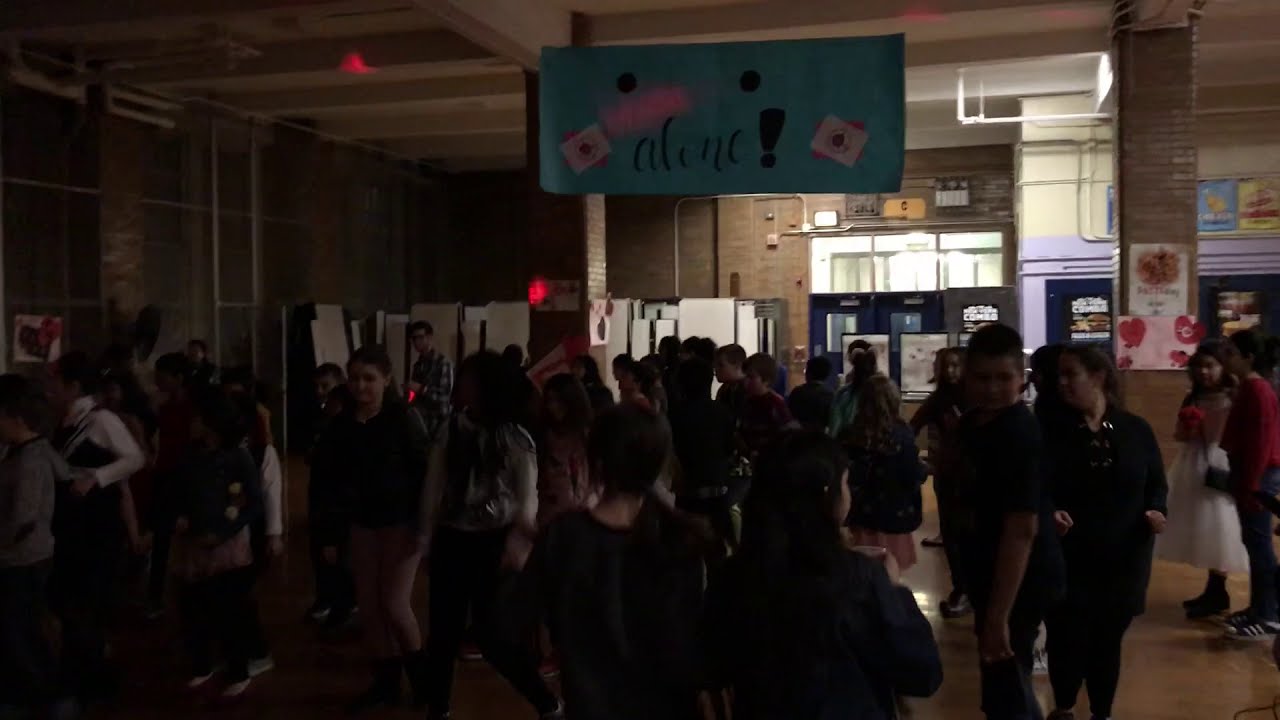In this dimly-lit indoor image, likely taken in a school, a large group of young people, possibly students, gather in the bottom half of the frame. The room is characterized by beige brick walls with supporting brick pillars reaching up to the ceiling. Despite the darkness, the upper-middle right side of the image has a light source, only partially illuminating the area. Central to the scene is a blue banner with the text "ALINI!" and other indistinguishable characters. There are red dots of light and various posters on the walls and doors, though their details are unclear. Some students appear to be holding objects, although the specifics are not visible. The overall ambiance is shadowy, with many details obscured by low lighting.